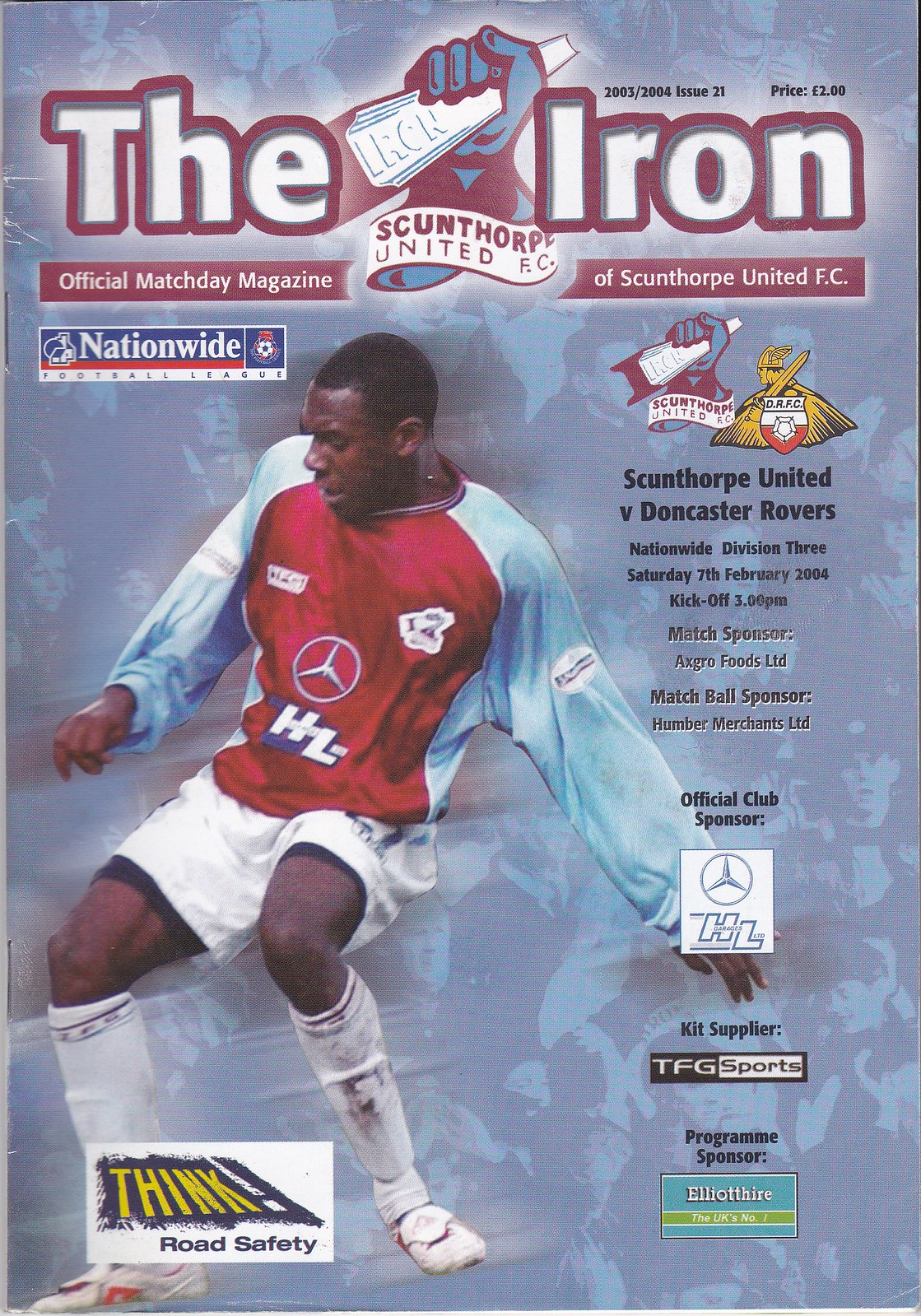The front cover of this soccer magazine prominently features an action shot of an African-American male soccer player who dominates the image with his dynamic pose. He is captured mid-game, bent over as if in the middle of an intense play. He wears a distinctive long-sleeve sweater with a red chest and blue sleeves, emblazoned with a prominent Mercedes-Benz logo in the center. His white shorts are paired with large white shin guards and socks, completing his athletic appearance.

The background blends into a blue hue, with a faded image depicting a crowd in the stands, enhancing the sense of a live game atmosphere. Above the player, bold white text with a red border announces "The Iron, Official Match Day Magazine of Scunthorpe United FC," and features a stylized graphic of a blue fist gripping a large iron rod, symbolizing strength and determination.

Additional details include information on the upcoming match: "Scunthorpe United versus Doncaster Rovers," scheduled for Saturday, 7th February 2004, with a kickoff at 3 p.m. The cover highlights various sponsors such as AXA Grow Foods Ltd, Humber Merchants Ltd, Elan Thyr, and the program sponsor "Think! Road Safety." A multitude of smaller sponsorship logos is scattered across the cover, adding to the vibrant, sports-centric design of the magazine.